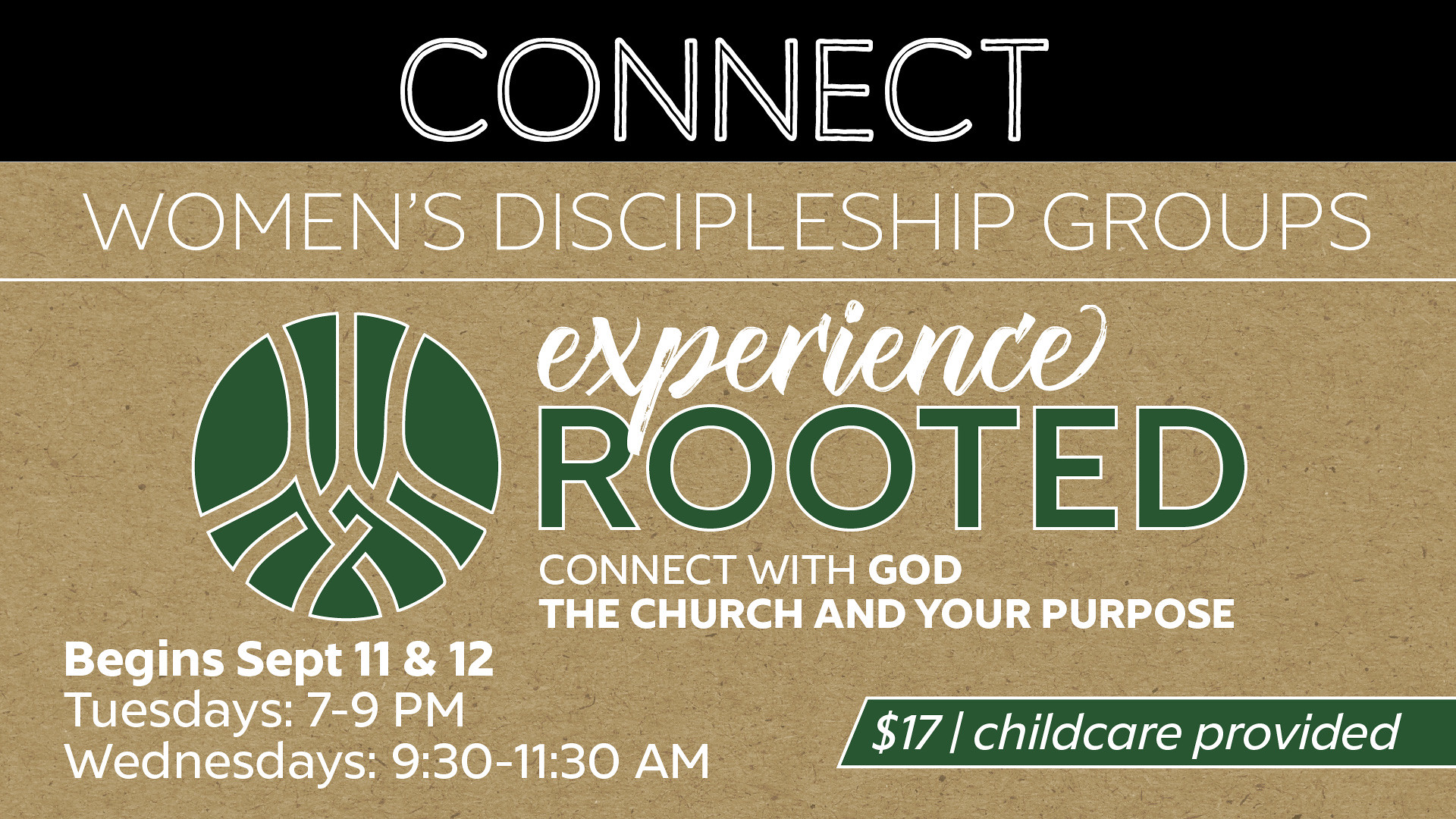The image is an advertisement for a church event. The top part features a black bar with "Connect" written in large white letters. Below this, the background transitions to a woody brown with darker brown spots, creating a rustic feel. In white font, it prominently announces "Women's Discipleship Groups," followed by a horizontal white line. In elegant cursive white lettering, the word "Experience" precedes green text that reads "Rooted." Adjacent to this, there is a round green symbol resembling tree roots. Further down, the text reads "Connect with God, the Church, and Your Purpose." On the left side, in white font, it details the event dates and times: "Begins September 11th and 12th, Tuesdays 7-9pm, Wednesdays 9:30-11:30am." A green box with white font highlights the cost and amenities: "$17, Child Care Provided."